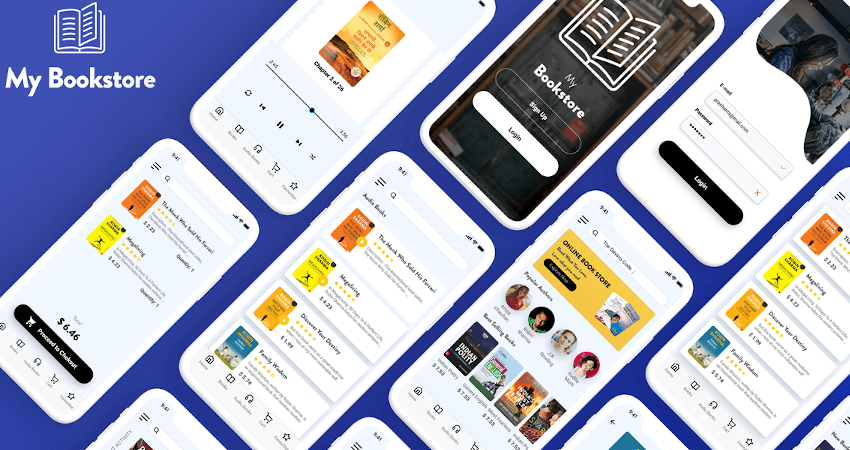The image is a vibrant and busy advertisement for an app called "My Bookstore." The background is a purplish-blue color, and in the top left corner, there's a white outline of a book with the text "My Bookstore" in white letters. In the foreground, several cell phones are arranged diagonally, showing different screens from the app. Each cell phone display highlights various features of the My Bookstore app: one screen shows a book titled "Chapters" with a progress indicator (e.g., 3 of 26) and media control buttons; another screen displays two books with prices listed (e.g., $6.46); others exhibit login/sign-up prompts, best-selling books, popular authors, and audio books. The overall design emphasizes the diverse functionalities of the My Bookstore app, showcasing it as a comprehensive digital platform for book lovers.